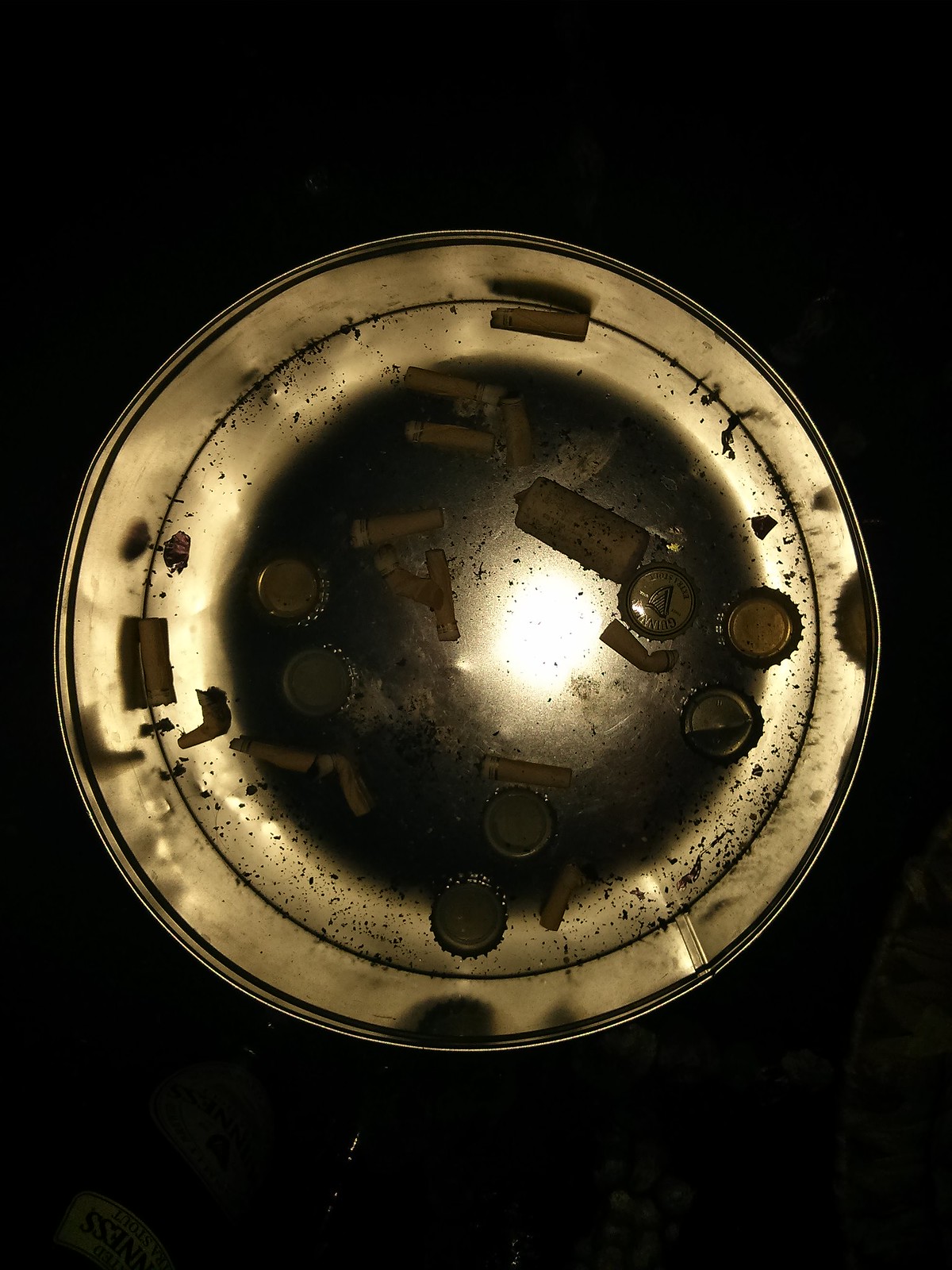This highly darkened photograph is taken top-down at night, capturing an illuminated metal container—likely a brass ashtray or a tin trash can—surrounded by pitch blackness due to the flash from the camera. The centerpiece is lit, revealing a mixture of debris: numerous soggy cigarette butts with their white tips and brownish-orange filters, several metal bottle caps—some featuring the Guinness logo—scattered within the container, and a notably long wine cork. The bottom of the container is partially visible and also shows accumulated dirt. In the lower corners of the image, faint, ambiguous shapes are present, adding a sense of mystery to the dim scene.